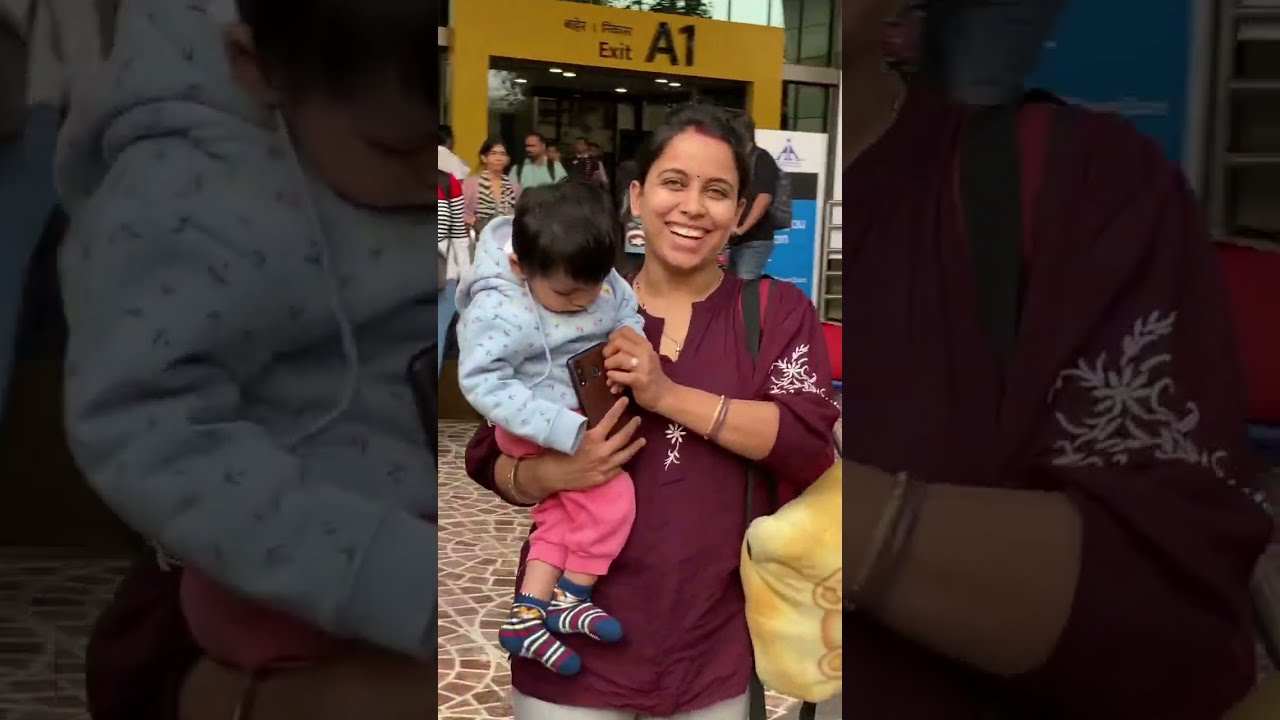In the center of this image is a smiling South Asian woman dressed in a maroon shirt featuring white floral patterns. The shirt has a slit down the middle of the collar, exposing a small rectangular area of skin, and its sleeves are pushed up to her elbows. She has black hair pulled back and is adorned with a gold bracelet on her right wrist. In her left hand, she is holding a small child who appears tired, dressed in a light gray hoodie, pink pants resembling bubble gum, and blue socks with red and white stripes. The child, with black hair, is reaching for the phone the woman holds in her right hand. Positioned in the bottom right of the image is a yellow bag.

The background shows a tan and brown tiled floor and an entryway towards the top, with a sign reading "Exit A1." Various people are visible in the background, wearing shirts in colors like magenta, blue, pink, and maroon. The setting suggests it might be outside a gate at an airport, and the style resembles a casual photograph, possibly taken as a screenshot from a mobile device app.